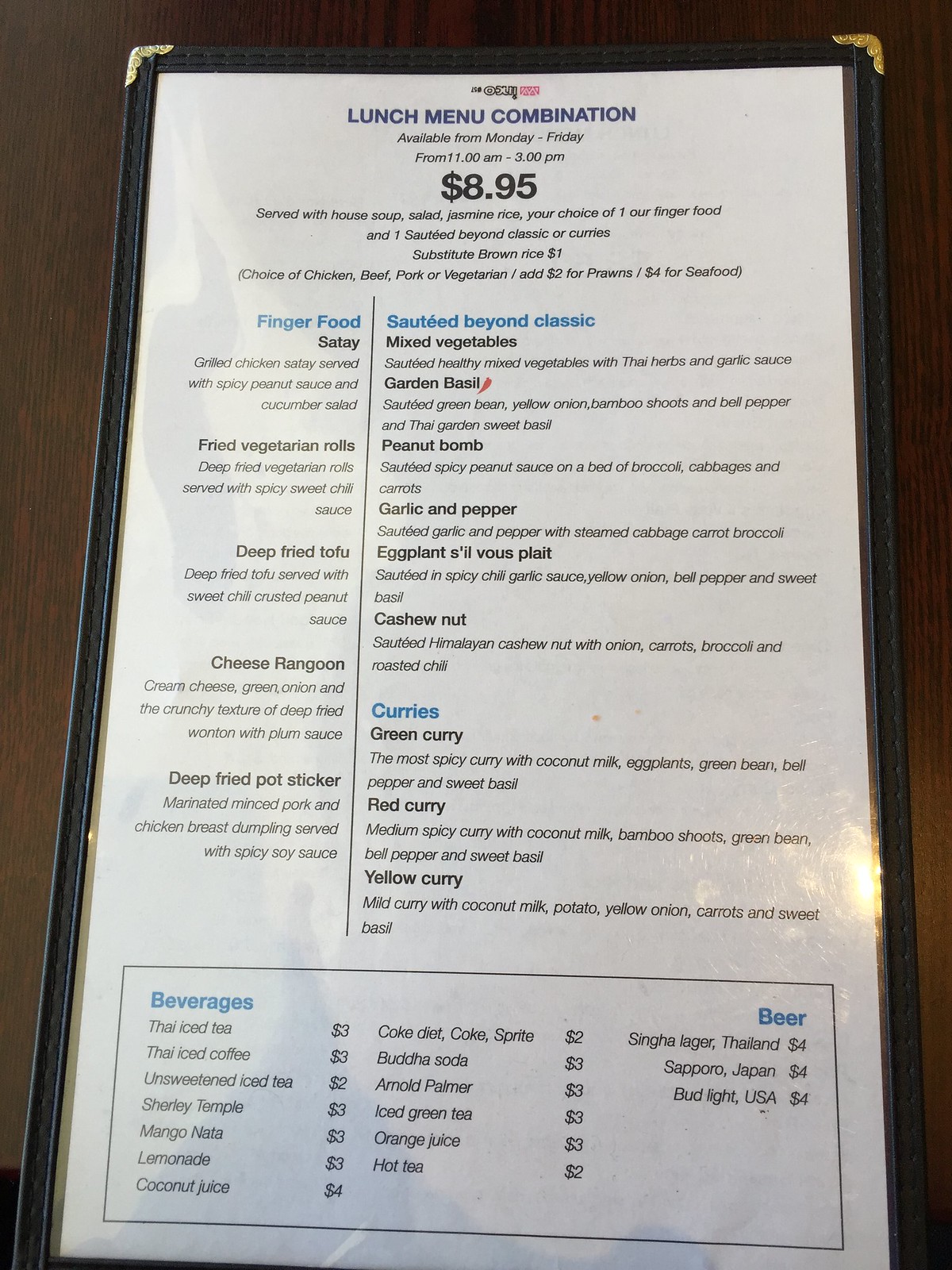A single-page lunch menu from a Thai restaurant is presented, featuring various categories of dishes and beverages available from Monday to Friday, 11 AM to 3 PM, priced at $8.95. The menu is divided into sections such as "Finger Foods," "Sautéed," "Curries," and "Beverages."

The "Sautéed" section, intriguingly named "Sautéed Beyond Classic," lists options like Mixed Vegetables, Garden Basil, Peanut Balm, and Garlic and Pepper. Under the "Curries" section, diners can find distinct varieties including Green Curry, Red Curry, and Yellow Curry.

For refreshing drinks, the selections include Thai Iced Tea, Thai Iced Coffee, and hot tea priced at $2. Unique offerings like Buddha Soda and Arnold Palmer are available for $3, while Sapporo Beer from Japan is listed at $4.

In the "Finger Foods" category, options such as Deep Fried Potstickers, Satay, and Cheese Rangoon are available, offering a delightful appetizer choice. Additionally, there is a note indicating a combination deal for $3.95, providing an economical option for mixing and matching these enticing items.